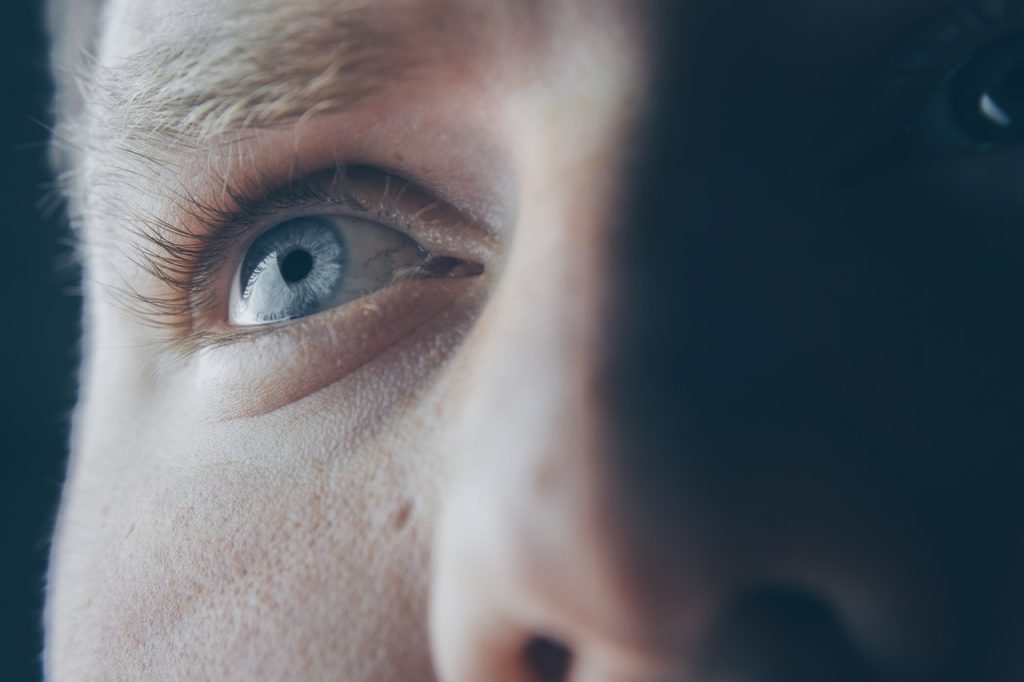This close-up color photograph captures the right side of a Caucasian man's face, with his sharp blue eye and light brown eyebrow as the focal points. Natural light illuminates half of his face, specifically his right cheek, eye, eyebrow, and the right side of his nose, creating a stark contrast with the shadowed left side. His light brown eyebrow appears fairly thick, extending over his expressive blue eye, which seems to reflect light, possibly from a nearby window. The detailed image reveals the pores of his skin under his eye, a small brown mole near the inner corner above the eyelid, and his long, brown eyelashes. His nostrils are noticeable but blurred due to the extreme close-up. The dark background emphasizes the highlighted features, adding depth to the image, which almost resembles a computer-generated graphic in its clarity and detail.